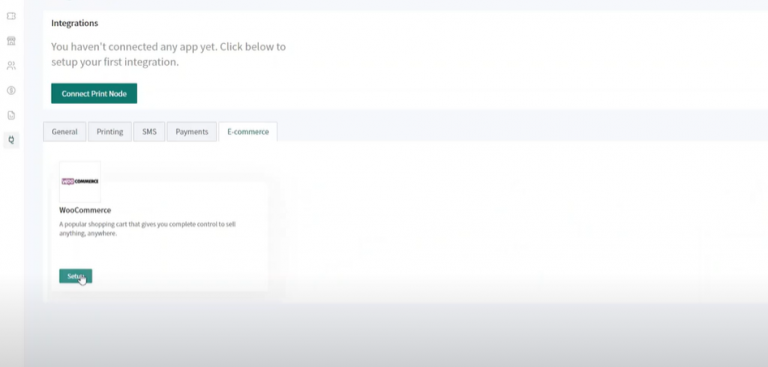This image appears to be a screenshot of a web-based application interface. On the left side, there is a vertical white sidebar featuring six gray icons arranged one below the other. To the right of the sidebar, the top section of the interface displays a prominent white search bar. On the top left corner of this bar, the word "Integrations" is displayed, and below it in large gray text, it reads, "You haven't connected any apps yet. Click below to set up your first integration."

Further down, a prominent green button labeled "Connect Print Node" is visible. Below this section, a series of tabs are aligned horizontally, labeled "General," "Printing," "SMS," "Payments," and "E-commerce," with the "E-commerce" tab currently selected.

In the main content area beneath these tabs, a box showcases a logo, accompanied by the text "WooCommerce." A body of descriptive text is placed below the logo, and another green button labeled "Send" is positioned at the bottom. The mouse cursor is seen hovering over this button.